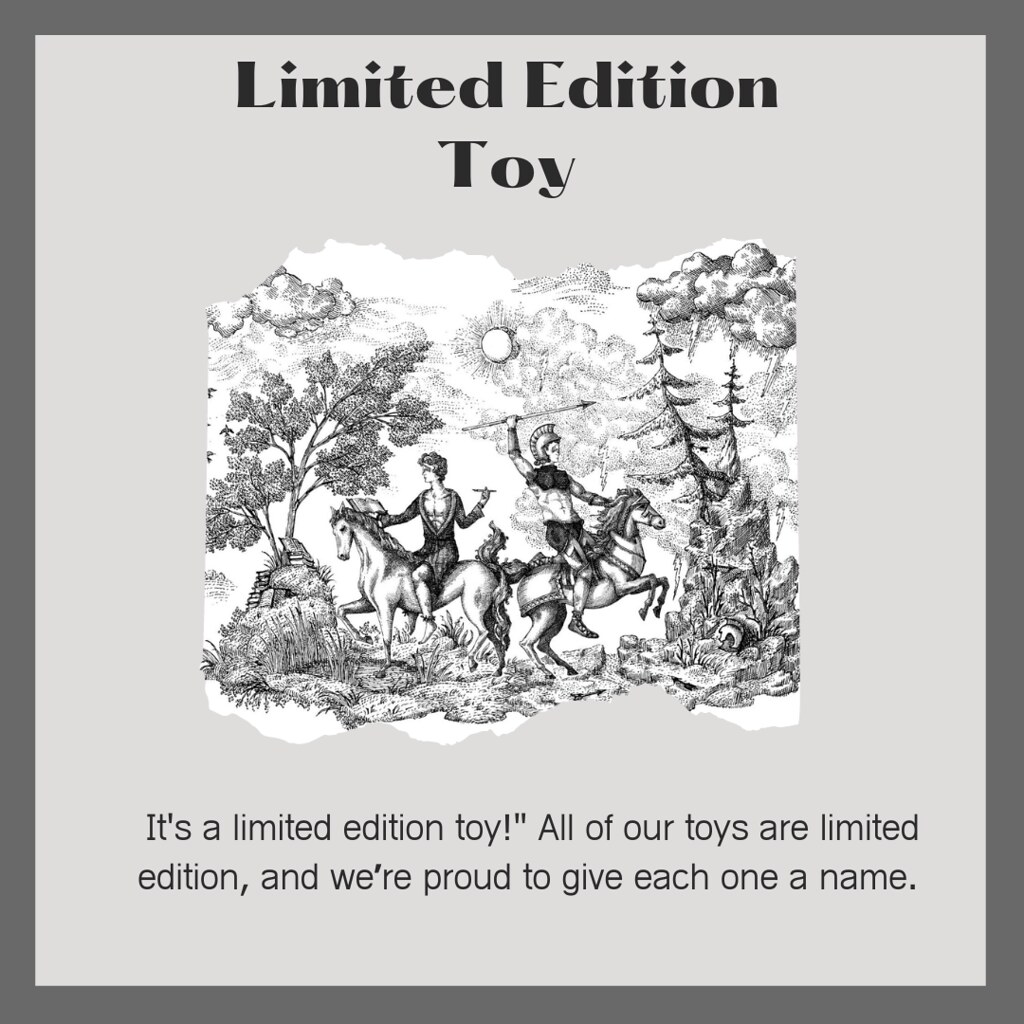This image is a detailed advertisement for a limited edition toy. It features a black and white artistic rendition centered against a light grey background, with a thick, dark grey border framing the composition. At the top, in a customized sans serif font, it reads "Limited Edition Toy," while the text at the bottom, in a smaller and lighter grey font, reaffirms, "It's a limited edition toy. All of our toys are limited edition and we're proud to give each one a name." 

The central illustration depicts two people riding horses. The horse on the left carries a rider who is reading a book and holding a pencil, suggesting an academic or contemplative persona. On the right, the other horse is rearing up, ridden by a person in armor holding a spear, embodying a warrior. The background includes detailed landscape elements, with a grassy hill and trees on the left, a rocky outcrop with more trees on the right, and a sun surrounded by clouds in the middle. Additionally, there are storm clouds above a mountain, enhancing the dramatic atmosphere of the scene.